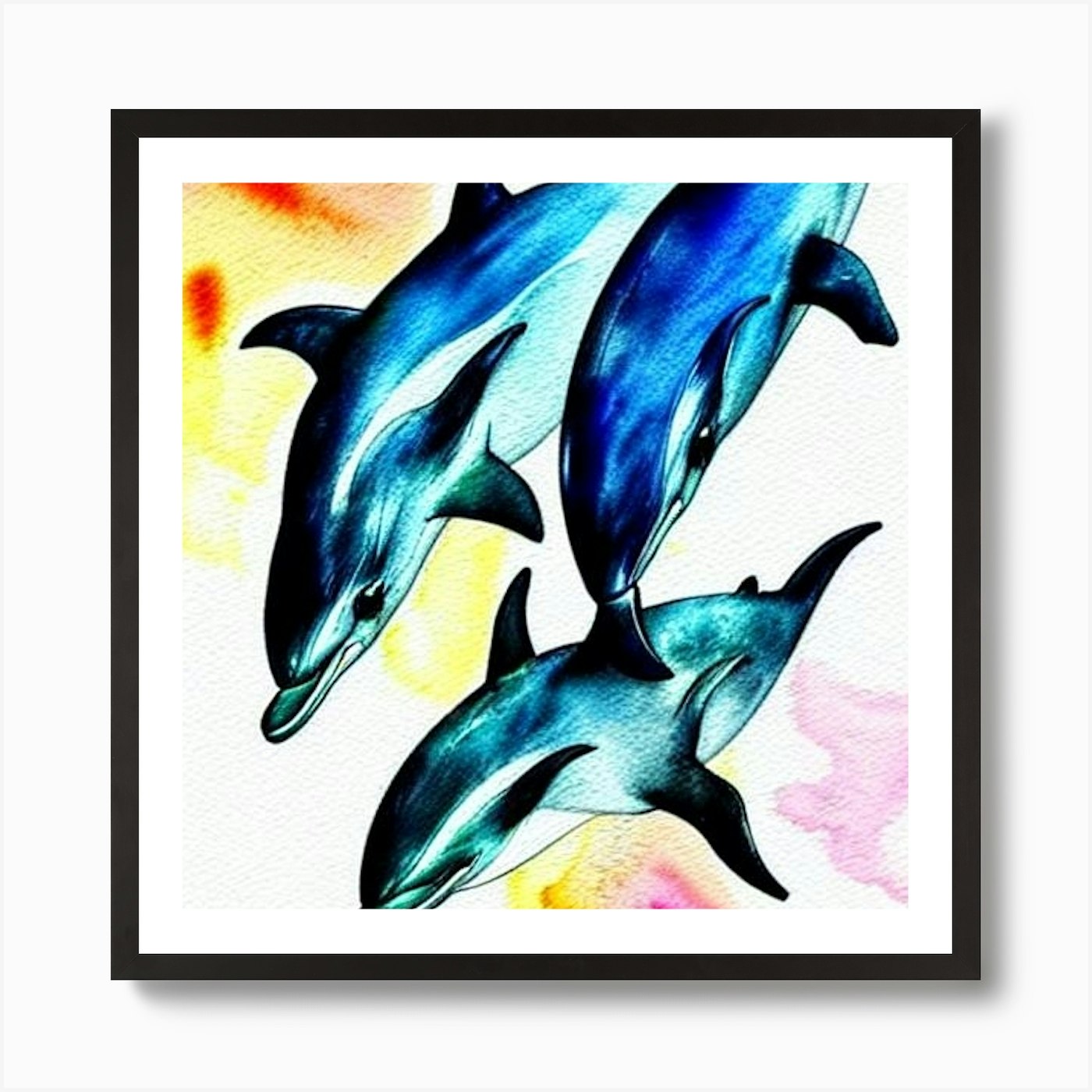The image is a color photograph of an art piece, most likely a watercolor painting, encased in a black frame. Within this frame, a white border made of highly textured paper surrounds the artwork. The main subjects are three dolphins swimming downward, varying in shades of blue, from aqua to dark blue, with black fins. One dolphin is noticeably larger, suggesting a family with a medium-sized dolphin and a smaller, possibly baby dolphin at the bottom.

The dolphins appear to have wire-like surfaces on their sides and display an unnatural alignment of fins, hinting at a possible AI-generated origin. Their faces feature small, pronounced noses, enhancing their whimsical appearance. The background is a vibrant blend of colors, with shades of orange, yellow, and white dominating the upper left corner while the bottom right corner showcases pinks, whites, and yellows, amidst numerous areas of plain white space.